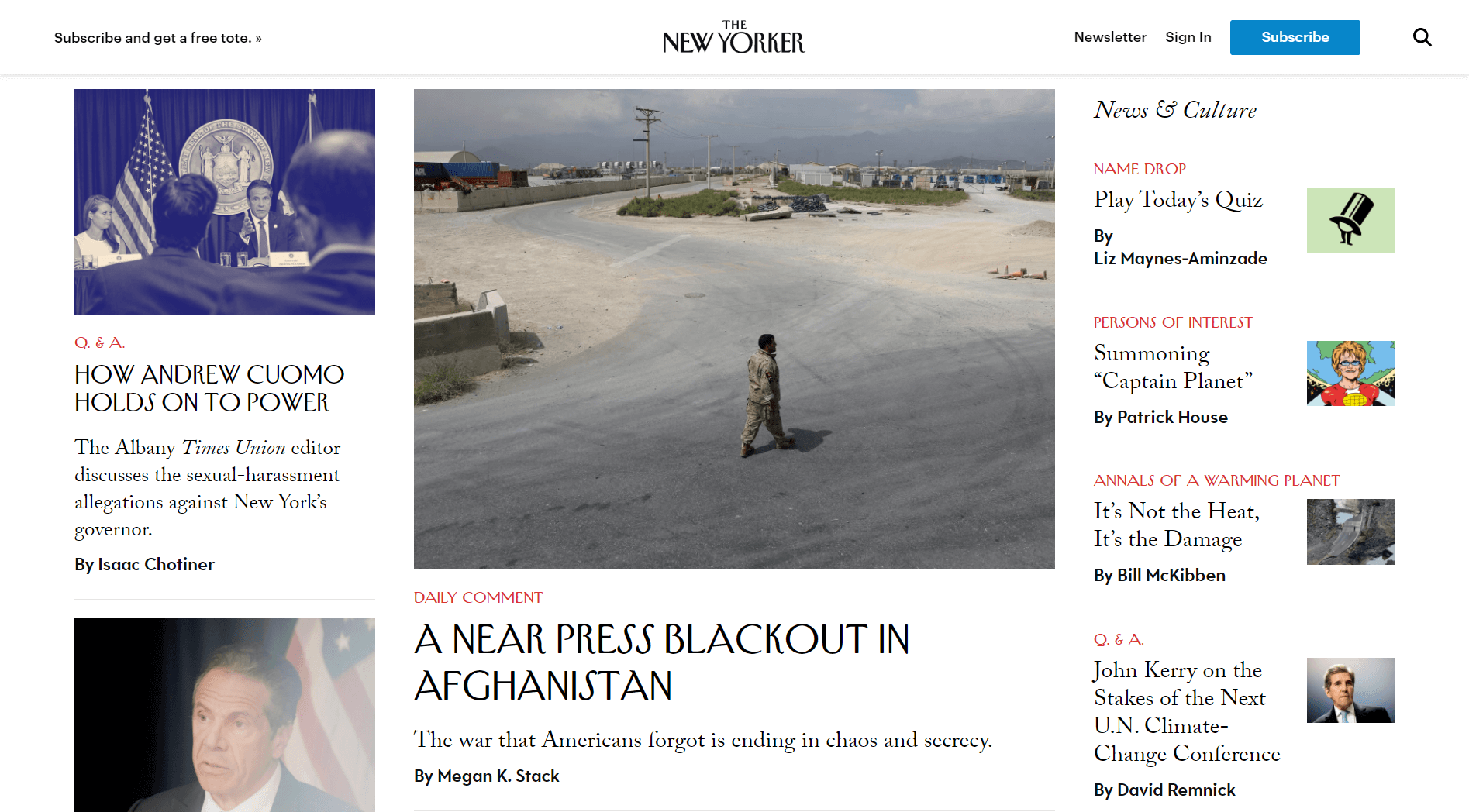This is a screenshot from the website of The New Yorker, featuring a white background and a layout of varied visual elements. At the very top is the header bar, which includes in the top-left corner a prompt that reads "Subscribe and get a free tote." Centered is the iconic logo and name, "The New Yorker." Moving across to the top-right, there are options labeled "Newsletter," "Sign in," a blue "Subscribe" button, and a search icon represented by a magnifying glass. This header is separated from the main content by a thin, light gray line.

In the left-hand column, a gray and white photograph shows rear-view shot of a crowd attending a speech delivered by a man in front of an official badge of office flanked by two American flags. Below this image, the text reads "How Andrew Cuomo Holds on to Power," followed by a snippet of the article and its byline. Below this, partially cut off, is a photograph of an elderly man turned to the left, with the U.S. flag positioned behind him to the right of the image.

The central focus of the page is the main article headlined "A Near-Press Blackout in Afghanistan: The War That Americans Forgot Is Ending in Chaos and Secrecy." The accompanying photograph depicts a desert-like camp scene, with a single figure walking along a road from the left towards the right.

On the far right-hand side is a column labeled "News and Culture.” It features various thumbnails: 
- "Play Today's Quiz" with a green thumbnail of a man in a top hat,
- "Persons of Interest: Summoning Captain Planet" with a thumbnail of Captain Planet,
- "Annals of a Warming Planet: It's Not the Heat, It's the Damage" with another thumbnail,
- "Q&A: John Kerry on the Stakes of the Next UN Climate Change Conference" with a thumbnail of John Kerry. 

This layout visually highlights recent and significant articles alongside visually engaging thumbnails, drawing readers' attention to a variety of topics at a glance.